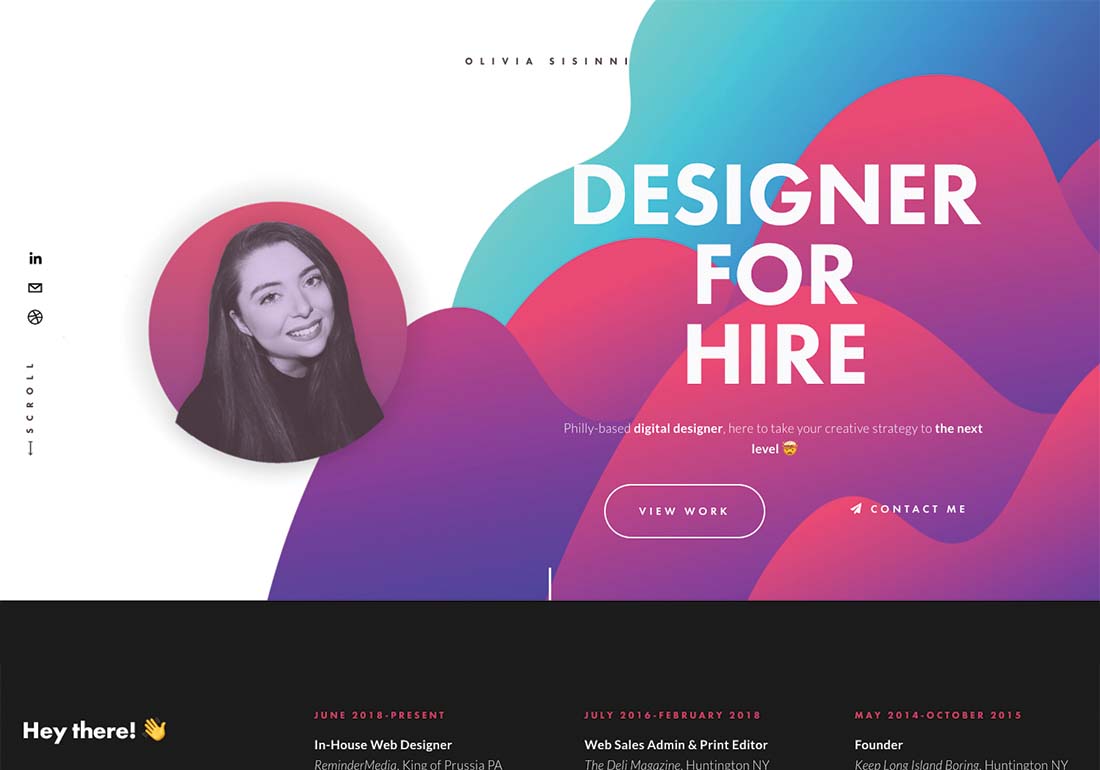This image is an online advertisement for a designer looking for work. It features a slightly rectangular, horizontally oriented layout. The background transitions from a white area on the left to a creatively designed right side that features a gradient resembling a sky at the top transitioning into blue, pink, and purple rounded forms reminiscent of hills.

On the left, in the white section, there is a circular photo of a young woman with long dark hair, smiling warmly at the camera. The background of the circle is pink. Above her photo, at the very top center in small letters, is the name "Olivia Sissini."

On the right side, bold white text reads, "Designer for Hire." Below this, in smaller letters, the text describes her as a "Philly-based digital designer, here to take your creative strategy to the next level," followed by an emoji.

Further down, an oval shape contains the text, "If you work." While someone seems to have interacted with this part of the ad, the details are unclear. Next to this, the phrase "Contact Me" appears.

At the bottom, there is a black bar; in the bottom right corner of this bar, white text says, "Hey there," next to an image of someone waving. There is additional text in this area, though its specifics are not detailed. 

Overall, this advertisement effectively presents Olivia Sissini as an approachable, talented designer ready to contribute to creative projects.